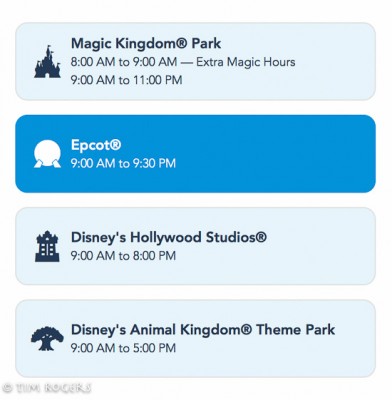This vertical image, slightly taller than it is wide, features a white background displaying what appears to be options from a cell phone interface. Spanning from left to right across the simulated screen are four rectangular buttons, each indicative of different theme parks. The first, third, and fourth buttons are highlighted in light blue, while the second button is shaded in medium blue, suggesting it is the currently selected option.

The first button features a black castle icon on the left, labeled "Magic Kingdom Park" in black text. Below the label, the operational hours are listed: "8 a.m. to 9 a.m. extra magic hours, 9 a.m. to 11 p.m."

The second, selected button displays a black crystal ball icon on the left and is labeled "Epcot" in white text, with the operational hours: "9 a.m. to 9:30 p.m."

The third button showcases a black tower-like structure on the left, labeled "Disney's Hollywood Studios" in black text. The time indicated is "9 a.m. to 8 p.m."

The fourth button bears a black tree icon, reminiscent of a Joshua tree, on the left side. It is labeled "Disney's Animal Kingdom Theme Park," with operational hours: "9 a.m. to 5 p.m."

Each icon and text label appears in black for visual clarity against the blue and white backgrounds.